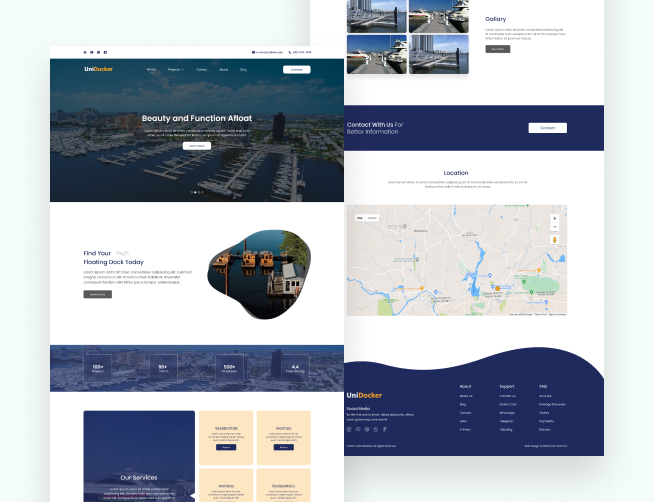A screenshot of a website called UniDocker, detailed as follows:

The top section of the page features the website's name with "Uni" in white and "Docker" in yellow. Despite the small and hard-to-read text, the main navigation options are not clearly discernible. The central area of the screen highlights two separate pages. The first page enthusiastically proclaims the "Beauty and Function of Float," drawing attention to its elegant design.

The second page showcases a picturesque marina filled with various boats and yachts, complemented by a banner that reads, "Find Your Floating Dock Today," emphasizing the website's purpose of assisting users in discovering floating docks and marinas. At the bottom, there is an assortment of numbers that are unreadable due to poor resolution.

In the bottom right-hand corner of the webpage, a blue box lists "Our Services," flanked by several options housed within yellow boxes featuring blue buttons. Adjacent to this section is a gallery displaying various images of boats docked in different marinas.

Further down, a "Contact Us" prompt encourages users to reach out for more information, situated next to an interactive map showing the company's location. Unfortunately, the footer of the webpage appears completely illegible due to resolution constraints. Overall, this website serves as a comprehensive guide for individuals seeking docking solutions for their boats.